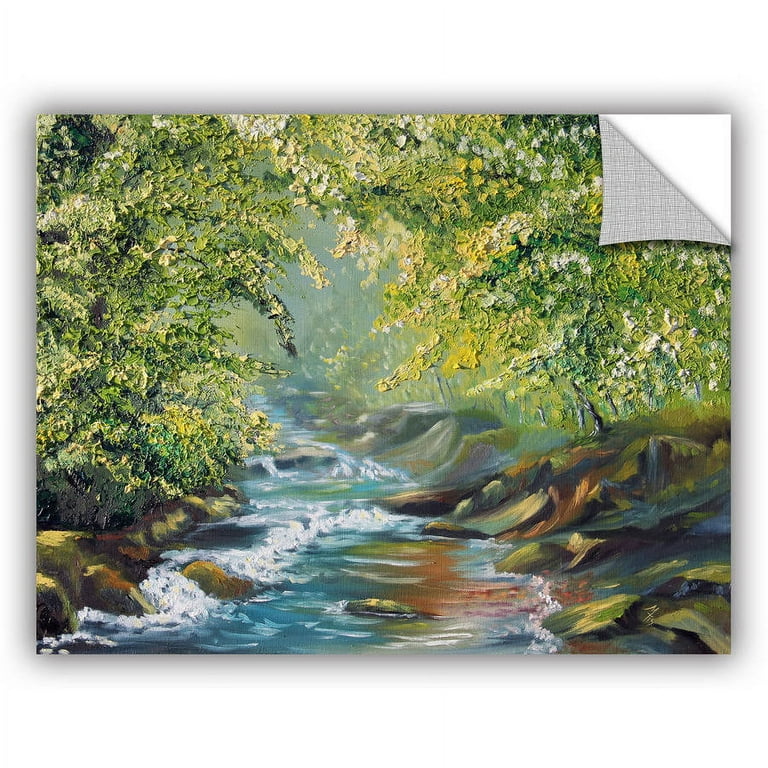The image showcases a professional piece of art, appearing to be either a painting or a drawing, depicting a serene natural scene. Dominating the center is a churning, babbling brook or stream, with white, frothy churns and blue hues, flanked by rocky shores on both sides. The rocks are a mixture of tan and gray, adding texture to the landscape. The scene is framed by lush green grass and trees, which exhibit a mix of green foliage, hints of yellow, and clusters of white flowers, suggesting a blossoming springtime setting. The tree branches and stems are rendered in shades of gray and brown, contributing to the depth and realism of the composition. The background hints at a distant forestry shrouded in gray, against a bluish sky. Notably, the upper right corner of the canvas seems to be peeling off, resembling a sticker, adding an unusual and intriguing element to the artwork. There is no text visible in the picture.